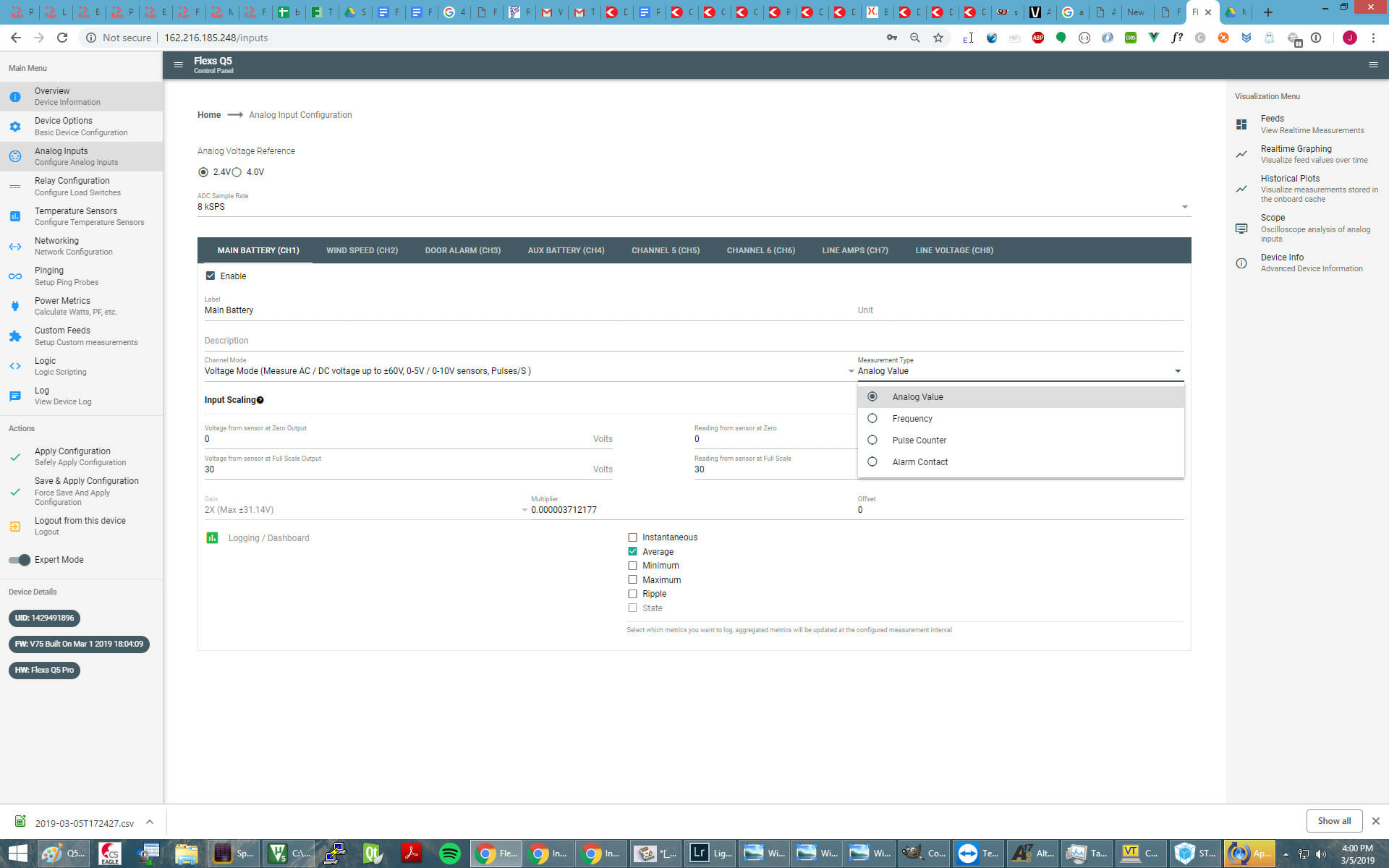In the screenshot, a webpage or application with a complex interface is shown, but the small text makes it difficult to identify. A light blue banner spans the top of the screen from left to right. Below the banner, multiple tabs or open applications are visible, though their details are obscured. On the top right corner, standard window control buttons—minimize, maximize, and close—are present. Beneath, a gray navigation bar includes left and right arrows, a refresh icon, and several other icons starting from the center and extending rightward.

On the left-hand side, a vertical column with a gray background displays black text, featuring some oblong boxes with white writing towards the bottom left. The main body of the screen is predominantly white, containing multiple fillable boxes for user input and making choices. This central section is encased by another gray border. Additionally, a right-hand column provides more selection options against a gray backdrop. At the bottom of the screen, mimicking the layout of a PC taskbar, there is a gray border indicating many currently open applications.